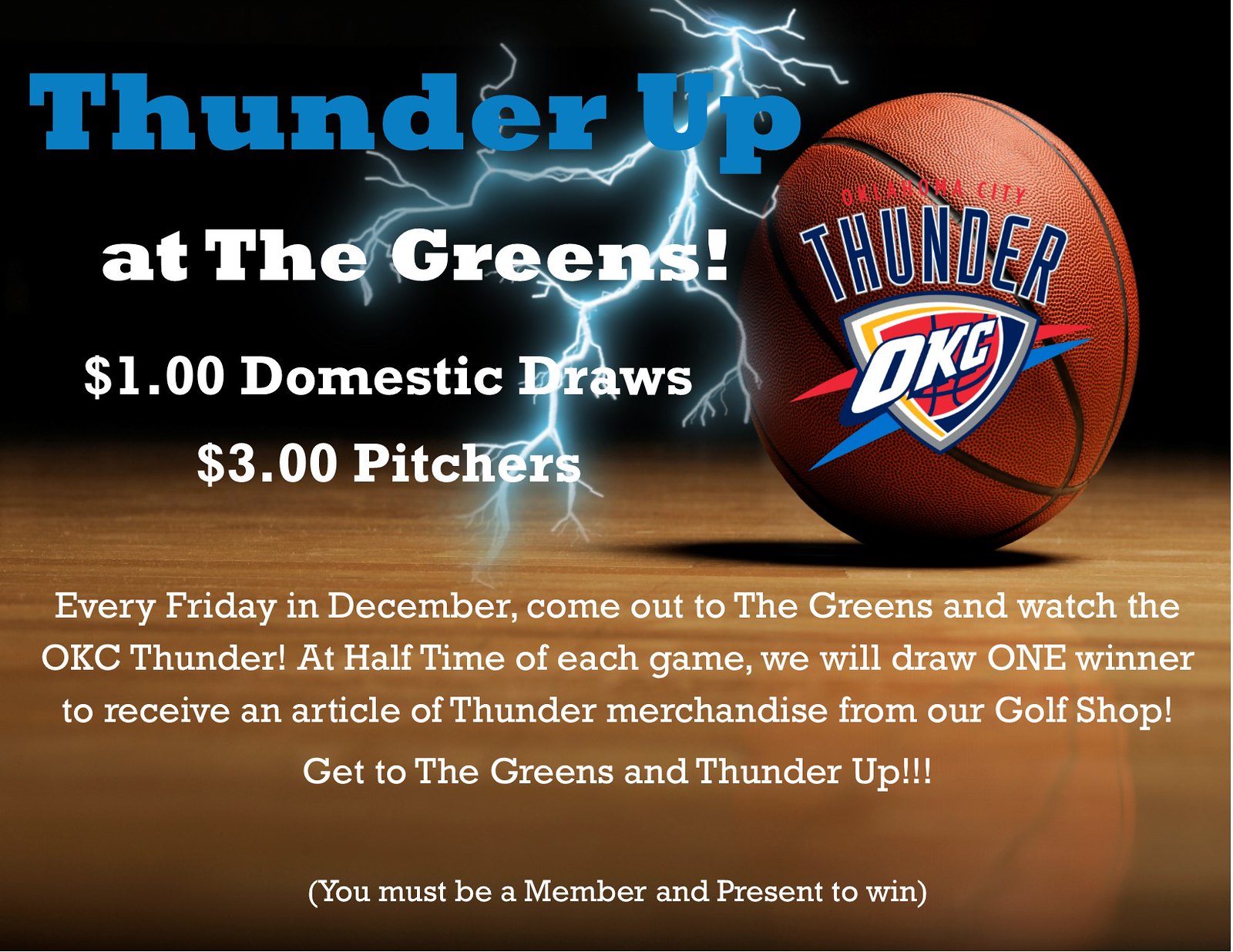The promotional poster is set against a black and brown background, with the brown resembling a wooden surface. At the top left in large blue letters, it reads "Thunder Up". From the center top of the poster, a lightning bolt strikes downwards to the middle of the image. To the right of "Thunder Up", there is a basketball featuring the Oklahoma City Thunder logo. The basketball has a shield-like emblem incorporating red, dark blue, yellow, white, and gray colors, with blue lettering that says "Thunder". Below the logo, a red triangle with white text spells out "OKC", and two streaks, one white and one blue, project from behind the triangle. 

On the left side of the poster, directly beneath "Thunder Up", in white lettering, it states: "At the Greens!". Below that, it offers "$1 Domestic Draws, $3 Pitchers". Further down in smaller print against the brown background, it reads: "Every Friday in December, come out to The Greens and watch the OKC Thunder. At halftime of each game, we will draw one winner to receive an article of Thunder merchandise from our golf shop. Get to The Greens and Thunder Up!" The message concludes with three exclamation points. At the very bottom, in parentheses, it mentions, "You must be a member and present to win."